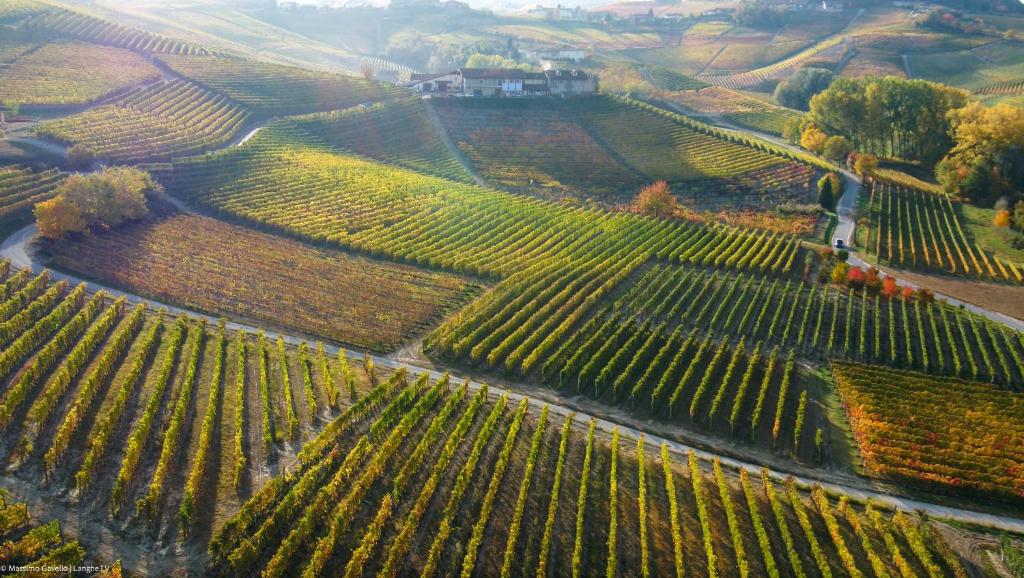This is an artistic aerial drawing of an expansive farmland with a patchwork of fields extending across rolling hills. The landscape is divided into numerous rectangular plots, showcasing a blend of fully-grown crops, harvested fields, and some yet to be planted. The crops are arranged in straight lines, diagonals, and various orientations. In the far background, under a haze that suggests sunlight, stands a large farmhouse complex. This complex appears as either a single large house or a tight grouping of buildings closely nestled together. To the right, there is a cluster of trees, while a prominent bush is evident to the far left. The intricate quilt of green, brown, and yellow fields is segmented by a few roads, adding structure to the picturesque scene.